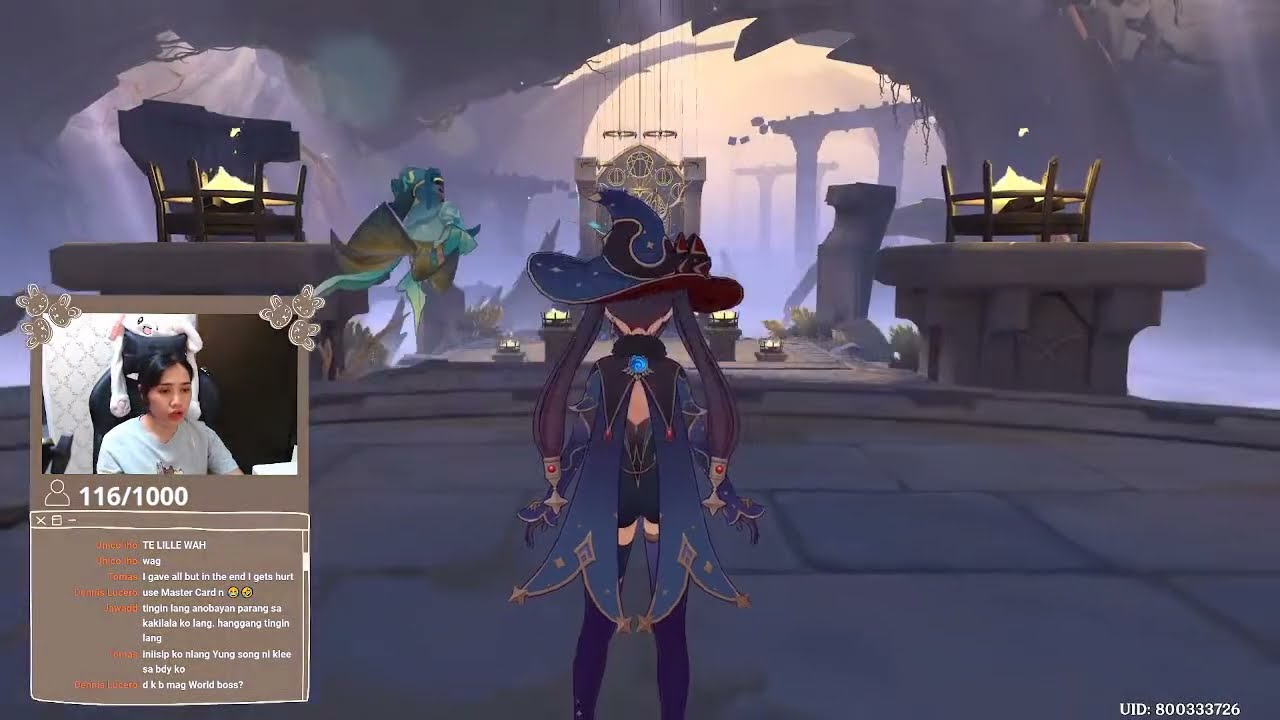The image shows a screenshot from a live-streamed video game on a platform like Twitch. On the left side of the screen, a female streamer with dark hair, wearing a light-colored (possibly blue) t-shirt, sits in a black gaming chair. Behind her, there is a white wall and a brown door, with some white lace décor visible. A streaming overlay box displays her live feed along with a chat box, containing orange and white text, partially obscured. Above the chat box, in the corners of her overlay, there are small graphics resembling kitten or bunny heads.

In the main part of the image, a female character, presumably the streamer’s avatar, stands out prominently. The character is dressed in a wizard-like outfit, complete with a large wizard's hat, a purple cape draping to the back of the knees, and dark blue short shorts. The character also wears pink or purple stockings. This character is positioned on a concrete bridge leading into a cave-like, magical fantasy environment. The setting features large gray rock formations and yellow-tinged sky, suggesting a high level or rooftop. The scene is dimly lit by two large green, flaming torches, and contains other green, soldier-like figures. At the bottom right of the screen, the game interface displays a UID: 800-333-726.